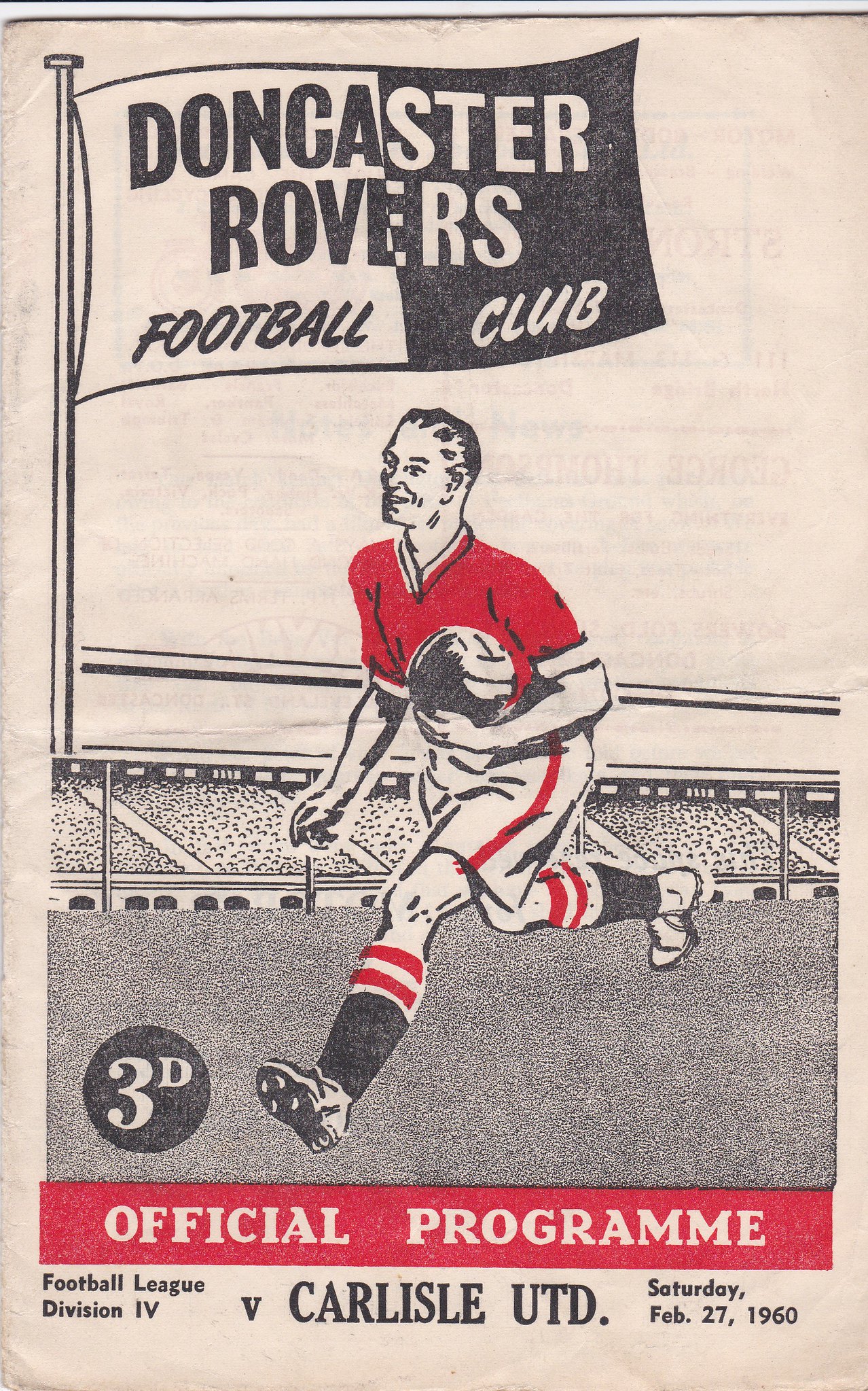The cover of the official program for the Doncaster Rovers Football Club depicts an illustrated scene. Dominating the image is a football player, dressed in a red v-neck shirt, white shorts with a red stripe down the side, and black socks adorned with white and red stripes. Oddly, he is running down the pitch, clutching the ball in his hand. Flying above in the upper left corner is a two-toned flag—white on the left and black on the right—proudly displaying "Doncaster Rovers Football Club." The background showcases a stadium packed with indistinct dots representing the crowd, emphasizing the full stands. In the lower left corner, a black circle encases the marking "3D." Below the illustration, a red rectangular band reads "Official Programme." Finally, at the very bottom, it states "Football League Division IV, versus Carlisle UTD, Saturday, February 27th, 1960." The cover has a vintage feel, printed in black and red ink on a slightly pinkish, aged paper, with reversed writing faintly visible from the opposite side.